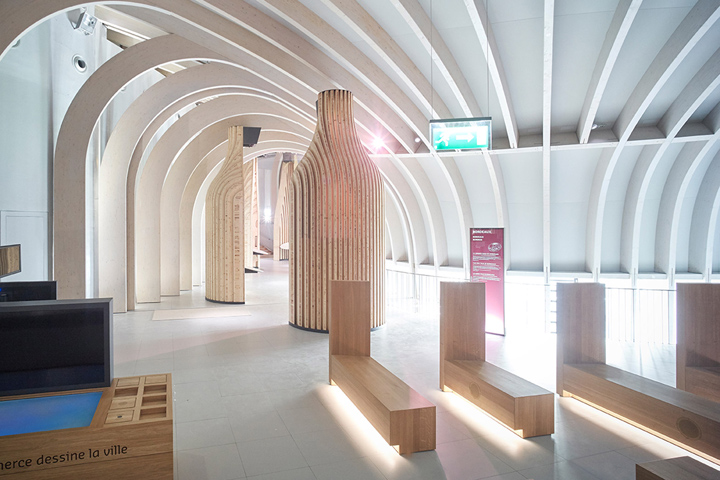The photograph depicts an interior space that appears to be a small art museum or exhibit room, characterized by its striking architectural elements and wooden furnishings. The room features vaulted ceilings composed of arched, white wooden slats that create a curved, tunnel-like effect. The lighting is primarily internal, as there are no visible windows, giving the space an intimate atmosphere.

Dominating the room are unique, large wooden sculptures reminiscent of giant milk bottles or wine bottles, intricately carved with layered patterns. These sculptures are accentuated by their polished wood finish, possibly pine, adding a warm, natural aesthetic to the room. 

The seating consists of minimalist, backless wooden benches with one end unusually tall, almost resembling backless church pews. These benches are strategically placed around the room, and some have soft lighting installed underneath, casting a gentle glow on the white tile floor. 

Additional details include a red informational sign installed near one of the seating areas, an exit sign affixed to the ceiling, and a small TV or monitor suspended by metal strings, suggesting a multimedia component to the display. There are also small black bookshelves and a couple of wooden tables scattered throughout the room, adding to the sense of a curated exhibition space.

Text appears in various parts of the image, including a smudged inscription in French on the lower left side, with legible words "Merci, Dessine, Love you," enhancing the artistic and cultural ambiance of the room.